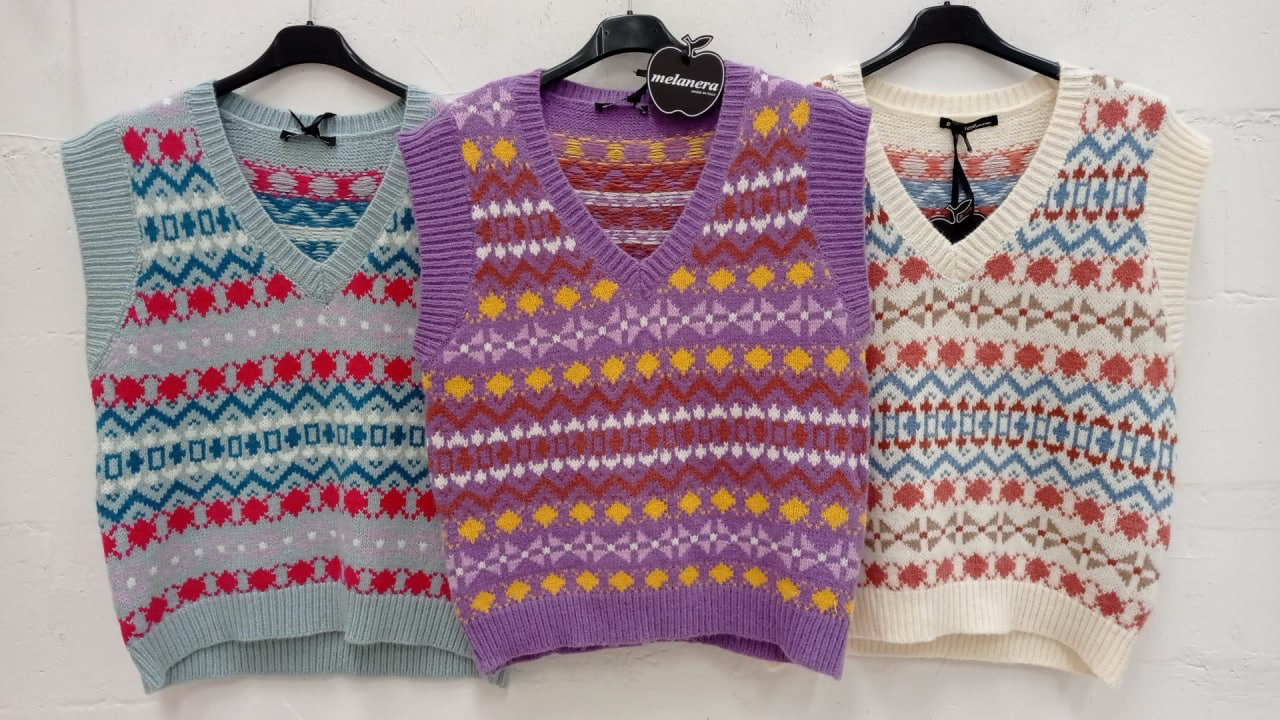This photograph features three uniquely patterned sweater vests hanging on black plastic hangers against a simple white wall background. The vests are arranged side by side with the one in the middle slightly overlapping the other two.

The sweater vest on the left is gray knit with a vibrant, intricate pattern consisting of alternating colors and designs: a line of red, white, green, and red interspersed with small white dots, continuing in layers of green, white, red, and then these detailed elements repeating across the fabric.

The middle sweater vest showcases a rich purple knit adorned with yellow diamonds and burgundy zigzag stripes. Delicate white flower-like details accentuate the pattern. A distinguishing feature of this vest is a black apple-shaped tag hanging near the neckline that reads "Melanera."

The sweater vest on the right is off-white with striking red diamonds and blue zigzag patterns running across its body, subtly accented by a light tan color. Each vest is characterized by its unique color scheme and pattern, emphasizing a blend of traditional knit designs and vivid colors.

These vests, likely displayed in a store, highlight the diversity in knitwear designs, making each piece stand out with its intricate detailing and vibrant hues.